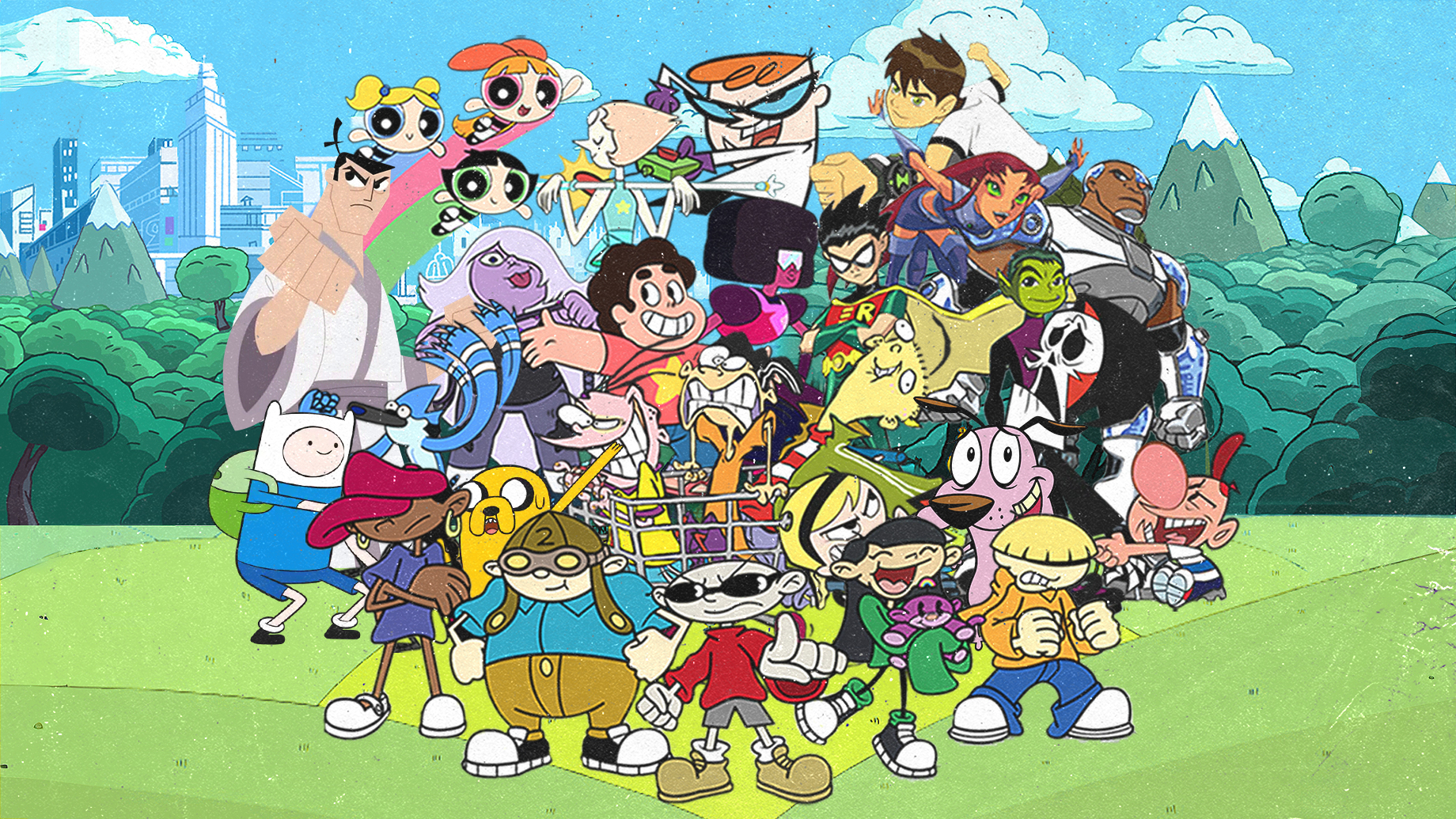This vibrant image of my childhood features a chaotic yet delightful ensemble of around 20 to 30 beloved cartoon characters from various animated series, reminiscent of a Cartoon Network extravaganza. Dominating the scene are the iconic Powerpuff Girls, each uniquely colored with Blonde-haired, blue-eyed Bubbles, black-haired, green-eyed Buttercup, and red-haired, pink-eyed Blossom. Amidst this nostalgic chaos, Dexter from Dexter’s Laboratory can be seen, possibly alongside his meddlesome sister Dee Dee. In the backdrop, idyllic scenery with grass, trees, mountains, and city structures under a clear blue sky frames the bustling assembly. The foreground is a playful mess of diverse characters piled atop one another, creating a captivating ball of animation. This includes characters spanning various ages and colors—children, old men, purple figures, a kid with sunglasses, a man in a cage, a baby crying, and a devilish character. Additionally, there's a notable purple dog, a woman acrobat, a man fighting, and a girl diving. This eclectic mix forms an imaginative snapshot, evoking the whimsical essence of animated adventures.